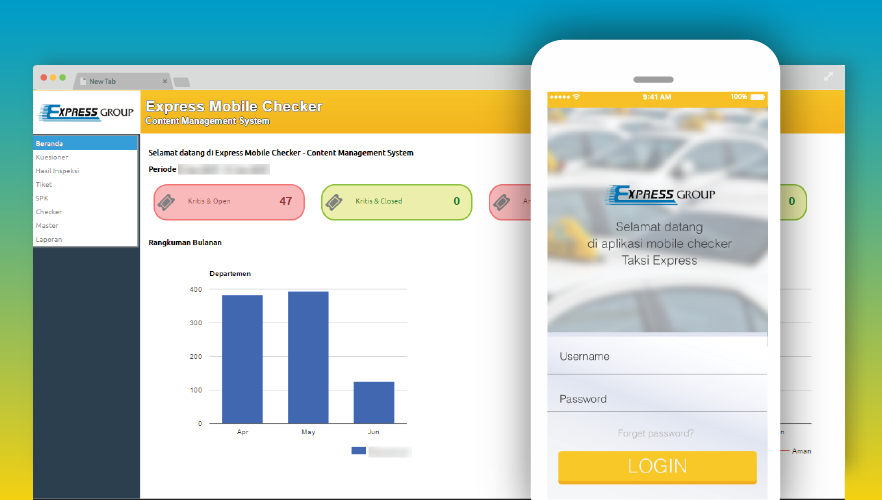This is a detailed horizontal image, reminiscent of a screenshot you might find on a computer or smart device. The background features a visually appealing gradient, starting with a teal blue at the top, transitioning to green, and finally to a yellow-orange hue at the bottom. Superimposed on this background is a website interface alongside an image of a smartphone.

The website overlay includes various elements. In the top-left corner, there are the familiar red, yellow, and green circular icons, often used to represent window controls. Adjacent to these icons is a new tab button, followed by the text "Express Group" and some vertically and horizontally oriented words in a different language. 

A prominent orange background section with white text reads "Express Mobile Checker, Content Management System." Within this section, there are various options enclosed in rounded rectangular boxes of different colors—red, green, and then red again. Below this, a bar graph is displayed, with numbers along the vertical axis and months labeled on the horizontal axis.

Overlapping this web interface is the image of a smartphone, which also displays the "Express Group" brand and the phrase "Selamat Datang Da Apalaski Mobile Checker Taksi Express." The smartphone screen shows fields for a username and password, along with a login button, creating a comprehensive visual of a web and mobile application interface.